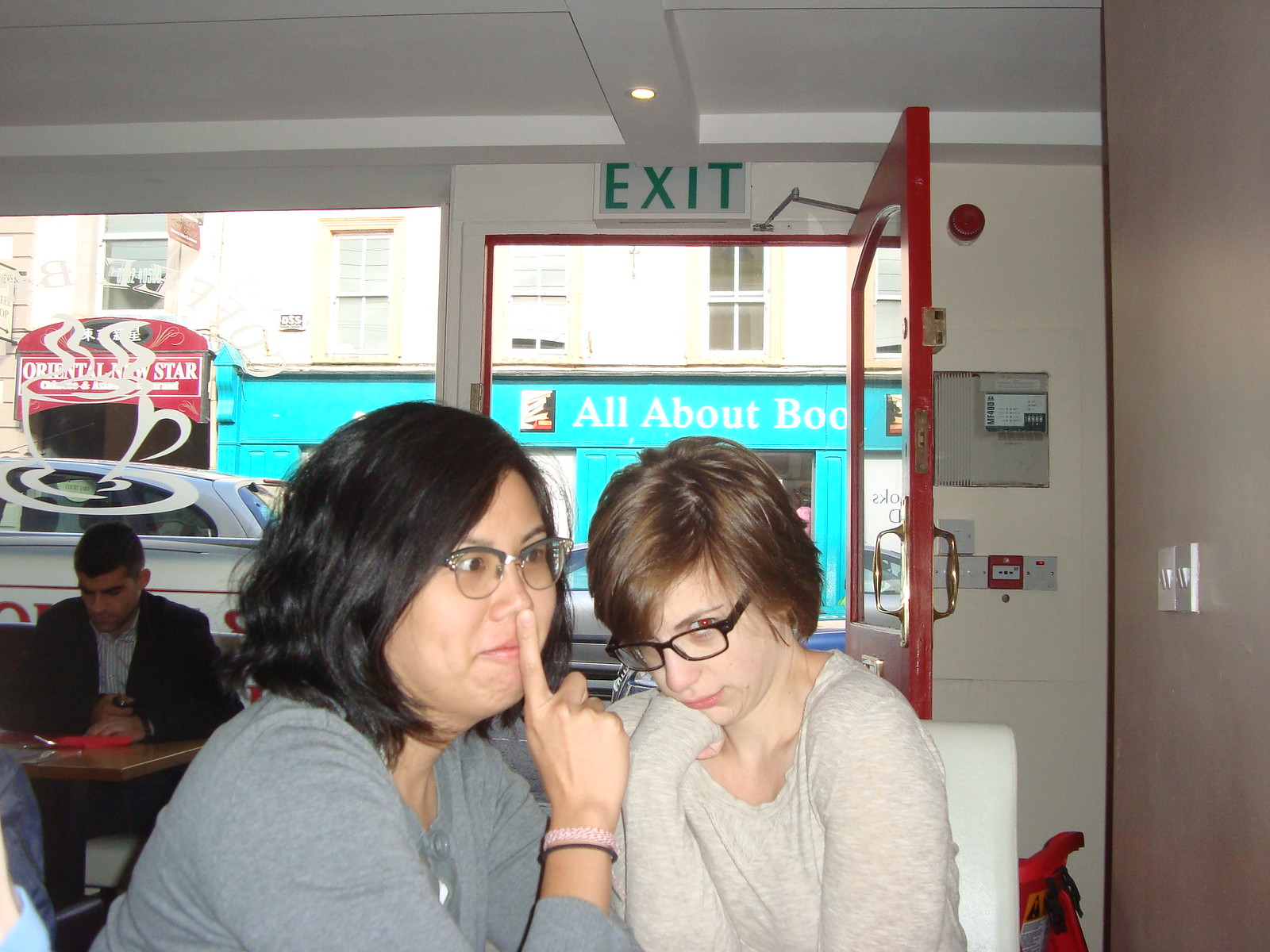This photograph captures a moment in a cozy café, featuring two women in the foreground, centered in the frame. The woman on the left is an Asian woman with shoulder-length black hair and glasses. She is wearing a greenish-gray long-sleeved t-shirt and is holding a finger to her lips in a quiet gesture, staring vacantly to the right of the frame. To her right sits a white woman with short brunette hair, also wearing black-framed glasses. She dons an off-white shirt, with her chin resting on her hand as she looks at the camera over the top of her glasses. Behind them, an open door with an "Exit" sign above it reveals a view across the street to a shop sign reading "All About Books". To the left of the women, a man in a business suit is seated at a table, working on a laptop. The café walls are light beige and white, with a window on the left side showcasing an outline of a coffee cup with steam rising from it. The setting suggests a tranquil atmosphere perfect for a quiet conversation or a moment of contemplation.